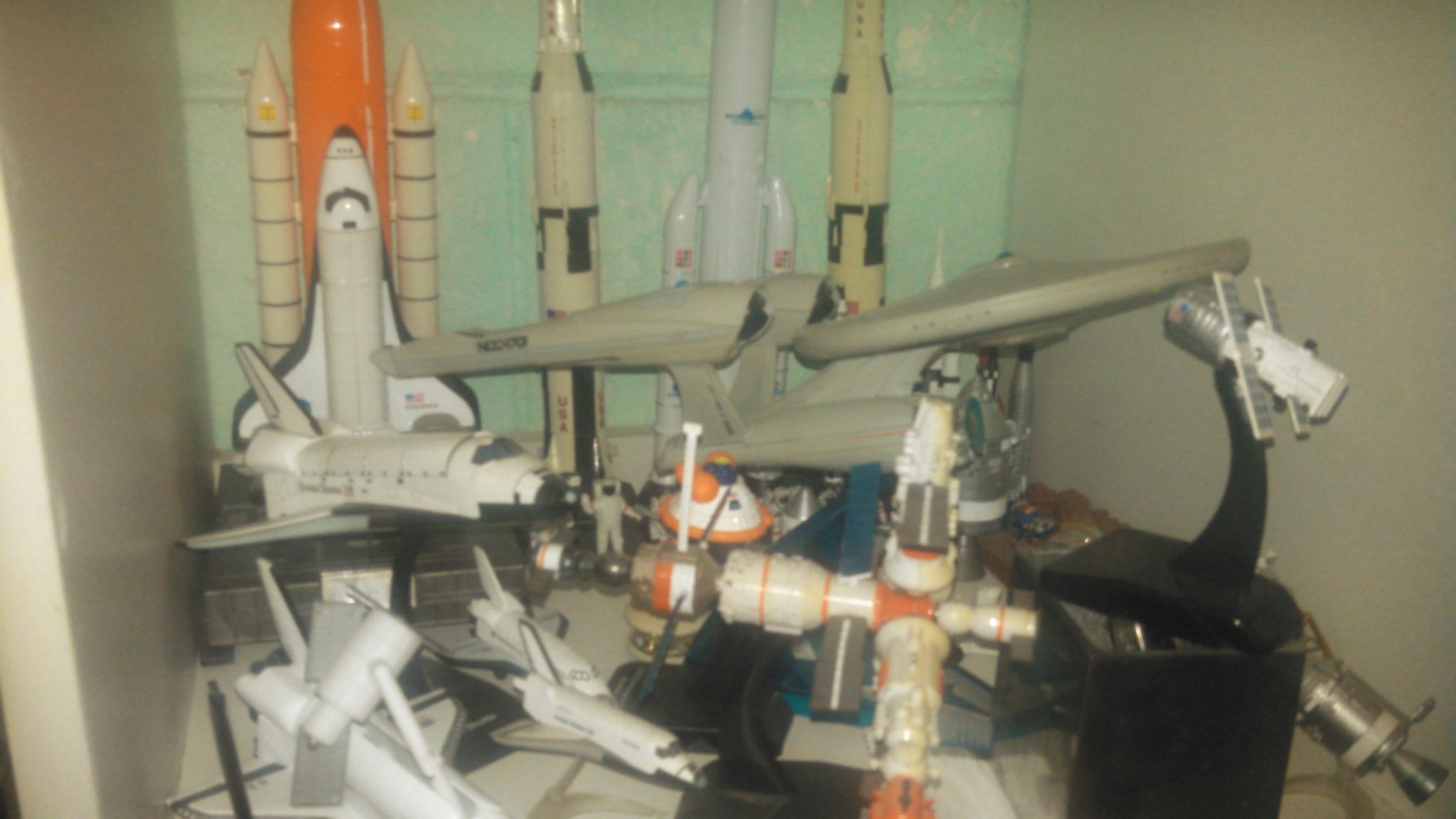The photograph captures a small, cluttered nook within a room, featuring an eclectic collection of model rockets, spacecraft, and satellites. The backdrop is a light turquoise teal blue wall, creating a contrasting setting for the predominantly white and gray scale models. Prominent among the models is a NASA space shuttle on the left, seemingly in flight and supported by a bracket. To the right, a satellite with two solar panels is held up by a black stand. In the center, a gray-toned model resembling the Starship Enterprise from Star Trek stands out with an oval-shaped front and angled back featuring large boosters. Additionally, there's another significant piece, an orange and white satellite, and the larger orange cylinder in the background adds to the variety. Scattered throughout are smaller, white spacecraft models, including what appears to be a white spacesuit figurine, all haphazardly placed yet forming an intriguing display against the green stone background.